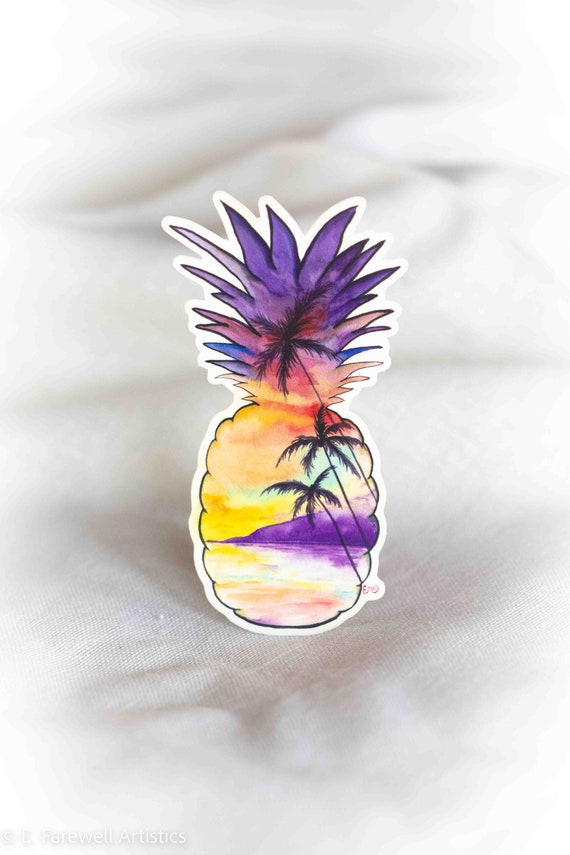The image features a detailed, artistic rendering of a pineapple-shaped sticker, placed centrally against a blurred white linen fabric background. The sticker itself is a vibrant beach landscape, transforming the shape of the pineapple into a tropical scene. At the base, hues of yellow, blue, purple, and red depict a serene ocean, merging seamlessly into a sunset sky towards the top. The sky transitions from yellow at the lower part to red in the middle and finally purple at the top. Two to three palm trees stretch diagonally from the right side of the pineapple shape toward the upper left, with a mountainous or hilly area illustrated in purple on the right side. The sticker is further embellished with a white penned outline of a palm tree extending from the leaves of the pineapple. At the bottom of the sticker, there is text reading "ENG," possibly a signature. The detailed texture and lines of the white linen fabric lightly frame the focused, colorful pineapple sticker, enhancing its visual appeal.